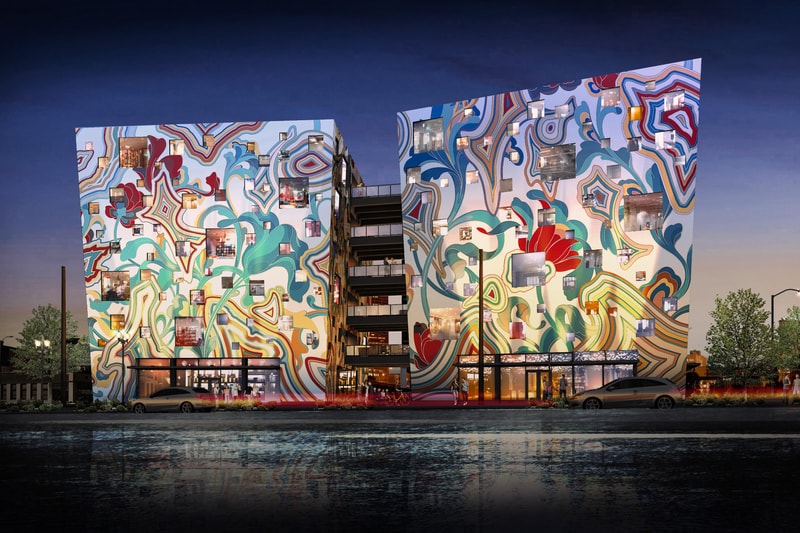The image captures a vibrant nighttime urban scene featuring a five-story modern building with two large, square sides adorned with extensive murals from top to bottom. These murals are brightly colored and depict a variety of geometric and wavy patterns, including concentric shapes in hues of green, blue, red, yellow, white, and orange. The two building sides are connected by five walkways that resemble stacked bridges, spanning from one side to the other on each floor. At the street level, the building has glass window entrances, and cars are visible parked in front, with the street itself appearing black and wet, possibly due to recent rain. The streetlights illuminate the area, and there's a striking visual of car taillights streaked out, suggestive of a time-exposure photograph. The sky above is a gradient of dark blue to black with hints of pink and orange near the horizon, adding to the rich ambiance of the scene. Trees are positioned alongside the building, enhancing the urban landscape.